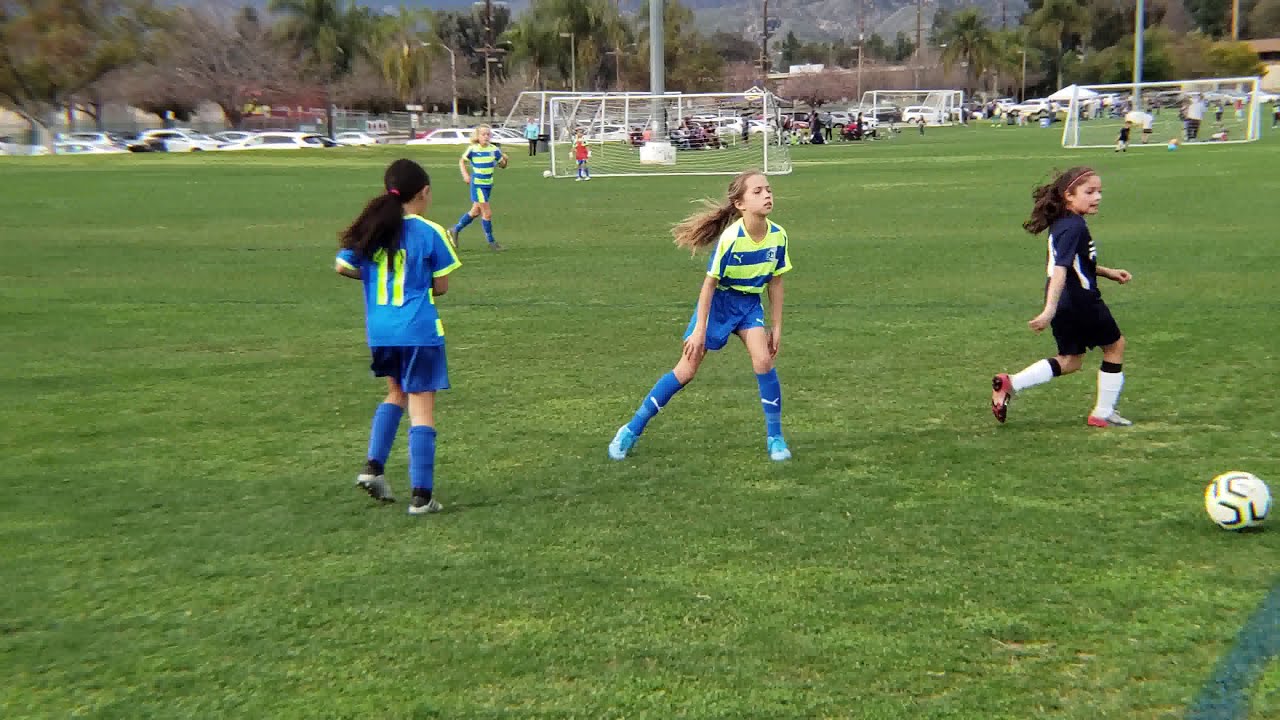This color photograph, in landscape orientation, captures a lively scene of young girls at a soccer practice within a park. In the foreground, three girls dominate the frame: the center player, approximately 8 to 10 years old, has long blonde hair and wears a blue and yellow striped jersey, blue shorts, blue socks, and blue tennis shoes. To her left, a girl with long dark hair, seen mainly from the back, sports a blue jersey with a yellow number 11, blue shorts, blue socks, and tennis shoes. On the right, another girl with dark hair pulled back by a headband is caught in motion, running after a soccer ball visible near the bottom-right corner of the image. She is dressed in a dark blue jersey and shorts, white socks, and red shoes. In the background, another girl in a blue and yellow uniform runs towards the foreground trio. Beyond the players, two soccer goals are visible, with several other children engaged in play. The surrounding area features a small crowd, cars parked in an adjacent lot, a brown building, and a line of trees that complete the picturesque setting. This image is a fine example of photographic representationalism, vividly depicting a typical day on the soccer field.